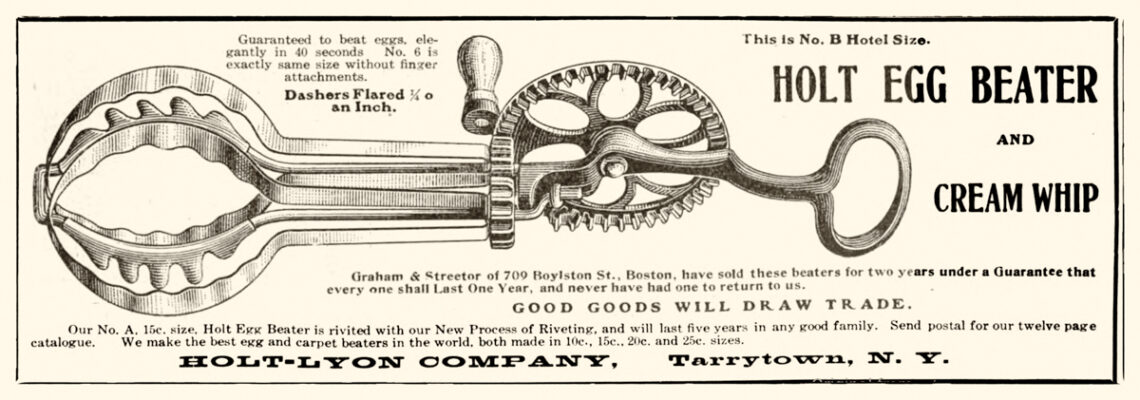This is a vintage advertisement for the Holt Egg Beater and Cream Whip, showcasing a detailed illustration of the hand-held mechanical device. The ad is rectangular, with prominent text on the right that reads "Holt Egg Beater and Cream Whip." The device depicted has a metal loop at the top, a wooden spinner handle in the middle, and a rounded bottom, featuring gear mechanisms that indicate its manual operation. At the top left of the advertisement, it claims, "Guaranteed to beat eggs elegantly in 40 seconds," and notes that "Number 6 is exactly the same size without finger attachments." The advertisement further mentions, "Dashers flared one fourth of an inch" and assures that "good goods will draw trade." Below the illustration of the egg beater, additional product details are provided. The bottom of the ad boldly lists the manufacturer as "Holt Lion Company, Tarrytown, New York."